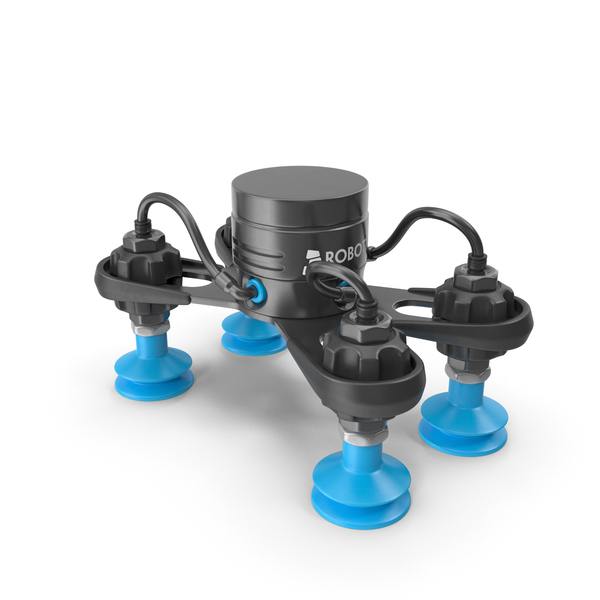The image portrays a sleek, black mechanical device that prominently features the word "Robo" inscribed in white on its central cylinder. The device has a round shape with four black circular attachments extending from it in an X-shaped configuration. Each attachment appears to function either as a top with rubberized sections or as a manual dial, hinting at adjustable settings. These attachments are interconnected to the central cylinder by an array of wires or tubes, emphasizing its intricate design. Below each circular attachment, the device is supported by blue structures that resemble feet or stands, possibly contributing to its stability. The base of each stand includes what look like silver nuts, followed by blue suction cup-like mechanisms, which might suggest a robotic function with potential up-and-down movement. All of these components are set against a clean, white background, highlighting the robotic and mechanical nature of the device, which could potentially serve multiple purposes, from floor cleaning to use in automotive or marine environments.